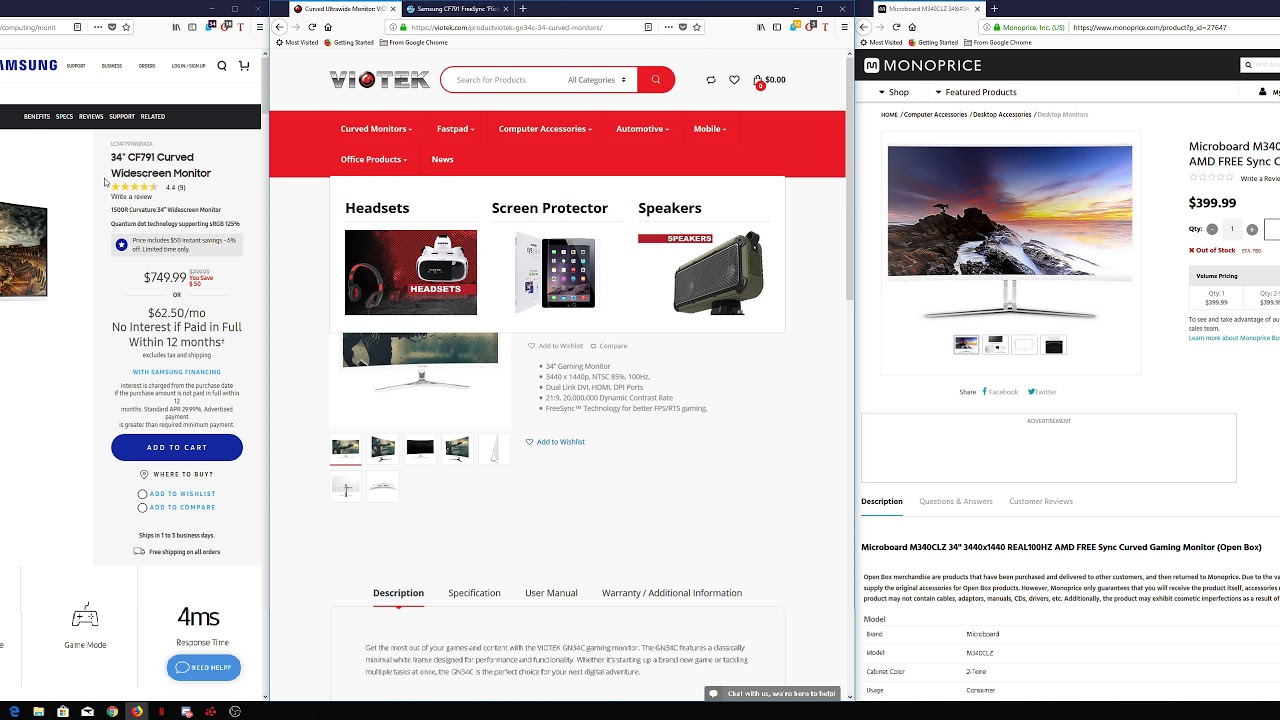The image depicts a large desktop monitor with at least three open tabs, suggesting the user is engaged in a detailed task, likely comparing prices or researching a specific product. The bottom of the screen features a black bar, probably the taskbar, filled with approximately ten different icons clustered on the left side. Among them, there appears to be the traditional 'E' icon for Internet Explorer, hinting at the use of older software.

The monitor has three primary tabs open:

1. **Left Tab**: Although partly cropped, the visible portion reveals a website displaying a Samsung product. This includes a photograph, a brief product description, and star ratings for customer reviews.

2. **Right Tab**: Partially visible and identified as the Monoprice website, it features a photograph, either of a television or a monitor, showing a picturesque mountain peak against a stunning sunset sky. Below the main image, there are several thumbnail images likely available for viewing different angles of the product and more details about the item, including its description and price.

3. **Middle Tab**: Fully visible and hosted on the Viotek website, which has a sleek, modern font with a distinctive red 'O' in the name. The top section includes a red-outlined search bar with a dropdown menu labeled "all categories" and a red button with a magnifying glass icon for initiating searches. Below this, a red navigation bar lists categories in white text, though they're too small to read in the image. The main content includes large photographs representing three categories: headsets, screen protectors (shown on a tablet), and speakers, the latter accompanied by a red banner. The white rectangle featuring these categories is partly concealing an underlying product image, which resembles the one seen in the left and right tabs.

Overall, the user appears to be comparing the same monitor or television across different e-commerce platforms, meticulously evaluating options to make an informed purchasing decision.